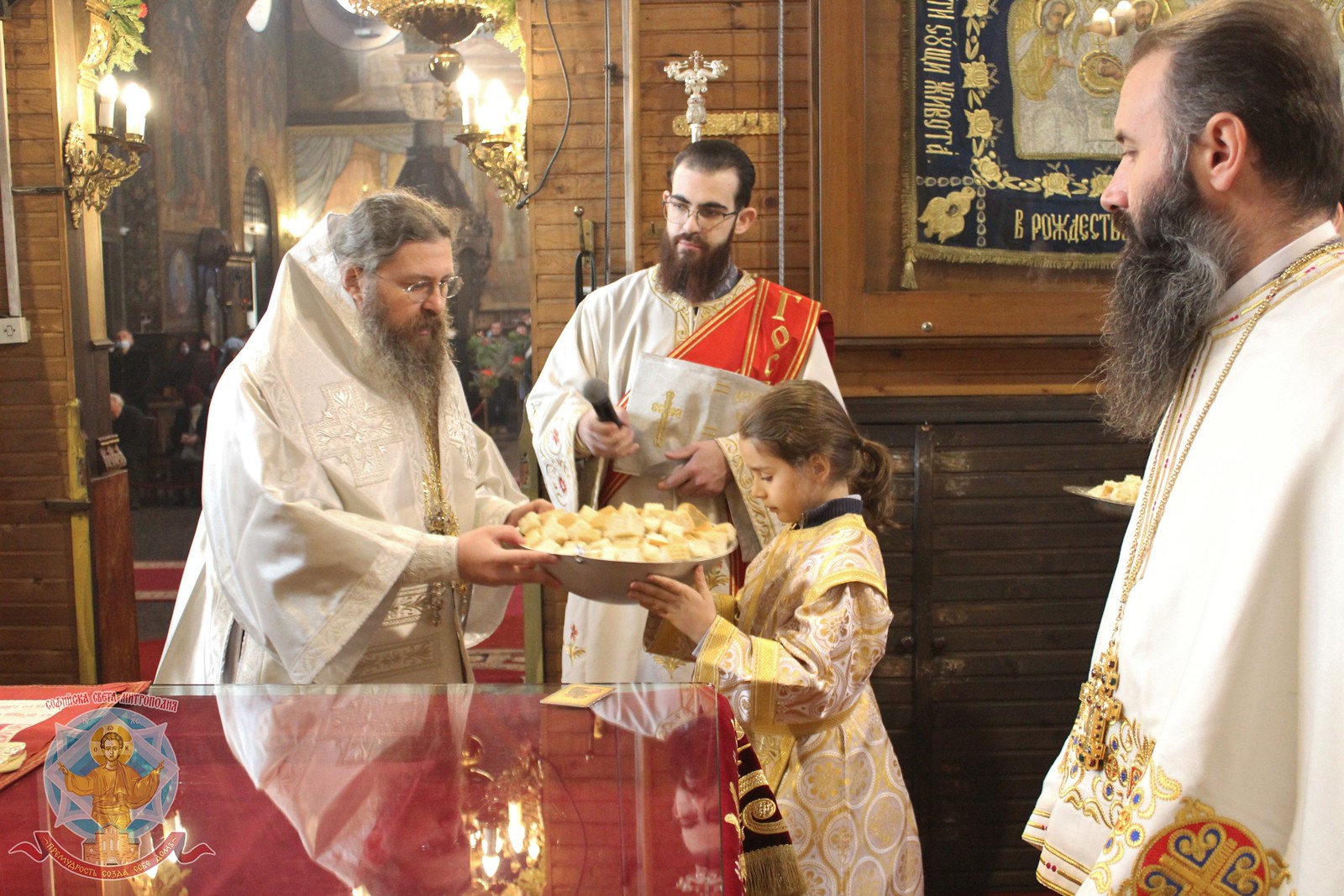In this detailed color photograph, captured inside an old building, likely a church, a ceremonial scene unfolds involving four individuals—all adorned in white and gold ceremonial robes, hinting at a Christian religious event. The backdrop features rustic brick and wood walls, enhancing the historical and solemn ambiance with hues of brown, gold, and white.

At the center of the image, two adult males stand; the one on the left cradles a large bowl filled with a food item, while the second man, standing slightly behind, looks towards him. A young girl, positioned in front of the bowl, reaches out with both hands, touching the food item as if about to receive it, signifying her involvement in the ritual. 

To the far right, an older man, distinguished by a prominent large gold crucifix hanging from his neck, observes the scene attentively.  His presence and the symbolic cross he wears underscore the Christian nature of the ceremony. The overall scene is framed by the warm, earthy tones of the wooden and brick interior, creating an atmosphere of reverence and tradition.